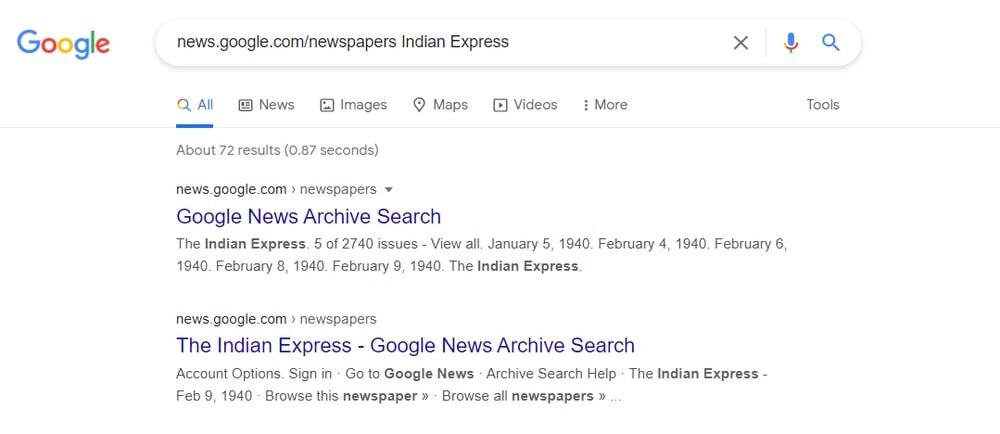The image displays a Google search results page. At the top left corner, the iconic multicolored "Google" logo is clearly visible. In the search bar, the query "news.google.com/newspapers Indian Express" has been entered. Directly below the search bar, there is a navigation menu offering options such as "All," "News," "Images," "Maps," "Videos," and "More," with "Tools" positioned towards the right.

The search results indicate around 72 results, found in approximately 0.87 seconds. The breadcrumb navigation reads: "news.google.com > newspapers > Google News Archive search," emphasizing the user's path within Google's news archive.

Further down the page, another breadcrumb trail is visible: "news.google.com > newspapers > Indian Express Google News Archive search," rendered in a bluish-purple color. Below this, there is an option to "Browse this newspaper" and a note stating “5 of 2740 issues” concerning the Indian Express, adding context to the extensive archive available for browsing.